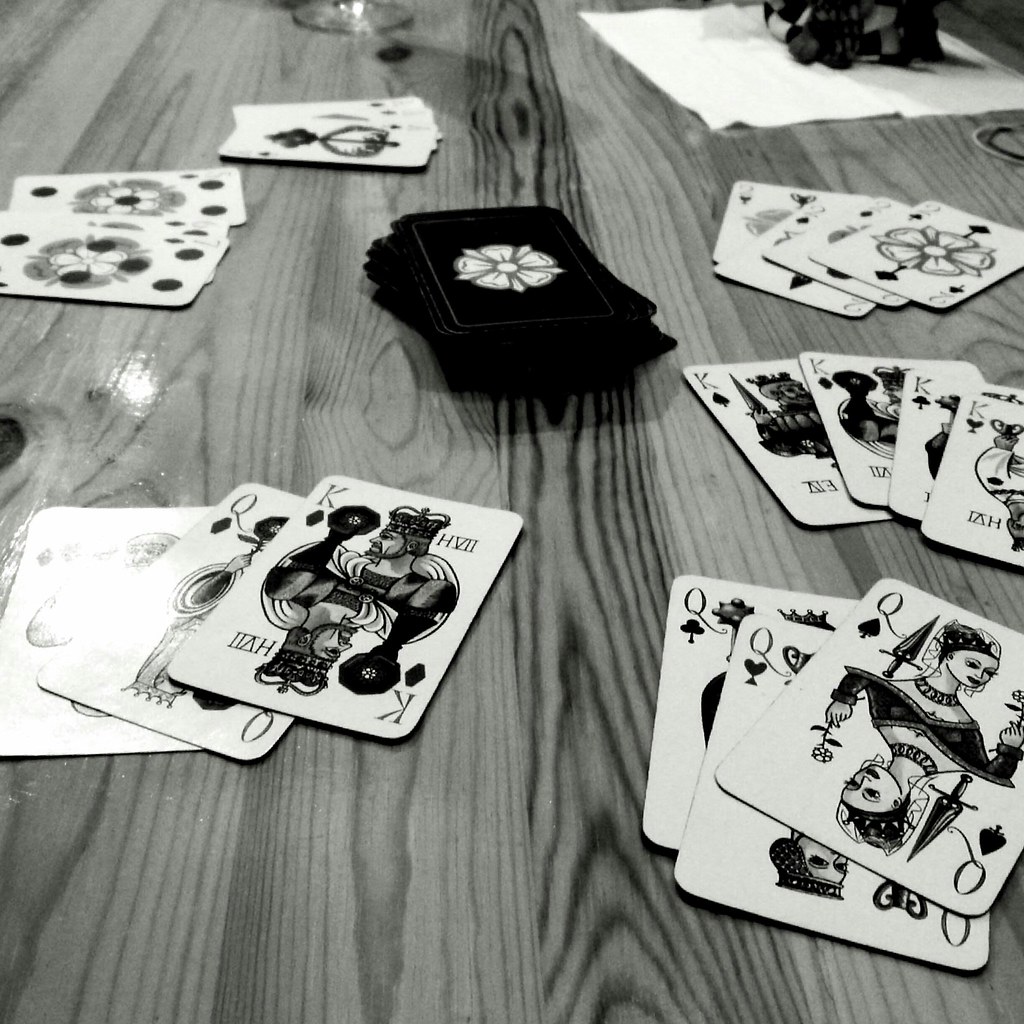This black and white photograph showcases an intricately arranged set of playing cards on a light-colored wooden table. The table itself serves as the backdrop, with distinct wood grain shading from upper center to lower center, lending a textured contrast that accentuates the overall composition. In the upper right corner, a paper napkin hosts various indistinguishable objects, adding a touch of casual realism to the scene.

The right side of the table displays an organized array of cards. In the right center, there are four cards: two of hearts, two of diamonds, two of clubs, and a faintly visible two of spades. Below this row, four kings are aligned: the king of spades, king of diamonds, king of clubs, and king of hearts. In the bottom right corner, the queen of clubs, queen of hearts, and queen of spades are stacked neatly, their unique, almost hand-drawn designs contributing an artistic flair.

The lower left corner reveals a mix of cards, where the king of diamonds, queen of diamonds, and possibly a jack of diamonds are slightly blurred. Centrally, more cards are scattered; some feature floral designs in their centers, enhancing the artistic intricacy. Furthermore, the backs of the cards, visible in the center of the image, exhibit a texture that appears almost velvety, highlighting the luxurious quality of this set.

This photograph captures not just the details of the cards, but their aesthetic value, emphasizing the artisan craftsmanship that makes this deck both visually striking and unique.